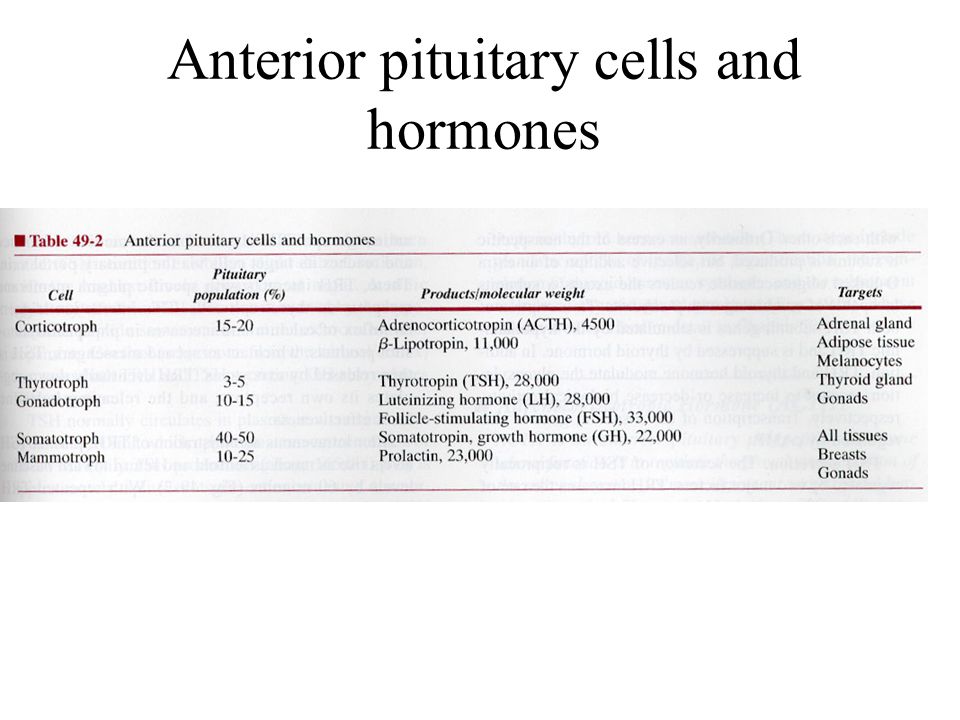The image depicts a partial page of a biology textbook, focusing on anterior pituitary cells and hormones, and appears as a screenshot pasted onto a plain white presentation slide. 

At the top of the slide, the title “Anterior Pituitary Cells and Hormones” is clearly printed. The picture itself is a black-and-white table accented with red horizontal lines of varying thickness, and is titled "Table 49-2" in red font, accompanied by a small red square on the left.

The table lists detailed information under four columns: "Cell," "Pituitary Population Percentage," "Products/Molecular Weight," and "Targets." Each cell type, including corticotroph, thyrotroph, gonadotroph, somatotroph, and mammotroph, is mentioned in the first column. The second column details their respective pituitary population percentages, ranging from 3-5% to 40-50%. 

The third column lists the products and molecular weights, such as adrenocorticotropin (ACTH, 4500), thyrotropin (TSH, 28,000), luteinizing hormone (LH, 28,000), follicle-stimulating hormone (FSH, 33,000), somatotropin growth hormone (GH, 22,000), and prolactin (23,000). The final column outlines the targets, which include the adrenal gland, adipose tissue, melanocytes, thyroid gland, gonads, all tissues, breasts, and gonads. The layout is crisply structured with thin red lines demarcating different sections of the table for clarity.